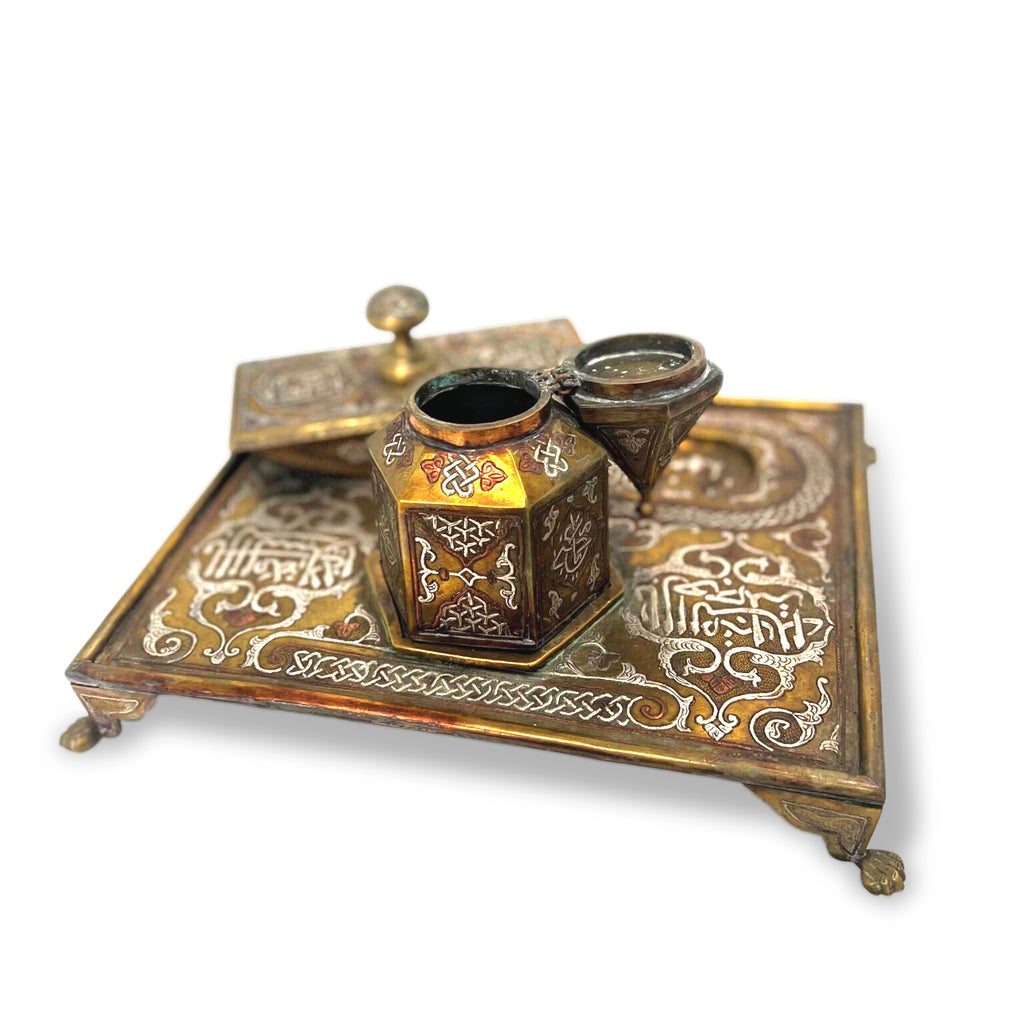The image portrays an antique, weather-beaten tray set against a white background, creating a stark contrast. The tray itself is light gold in color, accented with intricate, swirling white etchings and emblems that resemble both knot designs and rounded insignias. The flat surface of the tray is supported by ornate feet, each with three fingers extending towards the ground.

On top of the tray rests a hexagonal, crucible-like container. This golden container features a hinged cap that is propped open and tilted to the right. The cap has a circular knob at its end and exhibits signs of rust at the hinge. Behind the container, there is a slightly out-of-focus, copper-colored rectangular piece with a circular knob on top, suggesting another functional element. Subtle shadows cast to the right of the objects complete the composition, giving depth to what is likely a carefully staged stock image.